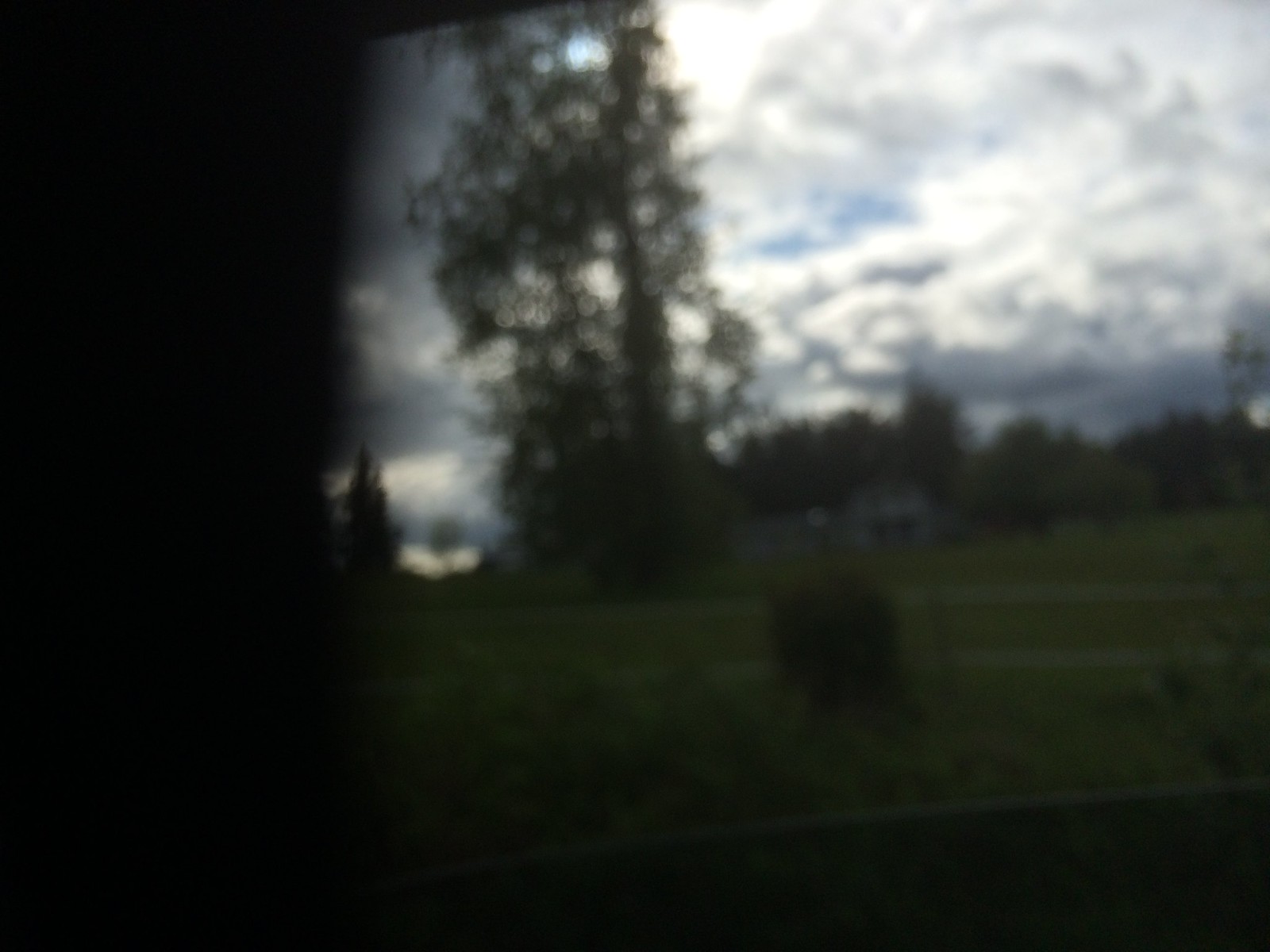This blurry photograph, likely taken from inside a building or vehicle due to the black borders on the left and bottom, captures a cloudy outdoor scene. Dominating the left side is a tall, slender tree, distinctly not an evergreen. In the far back left, a dark silhouette of evergreen trees is visible, forming a dense line. A large bush occupies the lower middle of the image, surrounded by patches of light green grass. In the background stands a white building, partially obscured by distance and light, and seemingly behind another fence. The overcast sky is predominantly gray with darker storm clouds on both sides, but there is a notable parting towards the center right where a patch of dark blue sky peeks through. The photograph is characterized by its haziness, making it challenging to discern finer details.